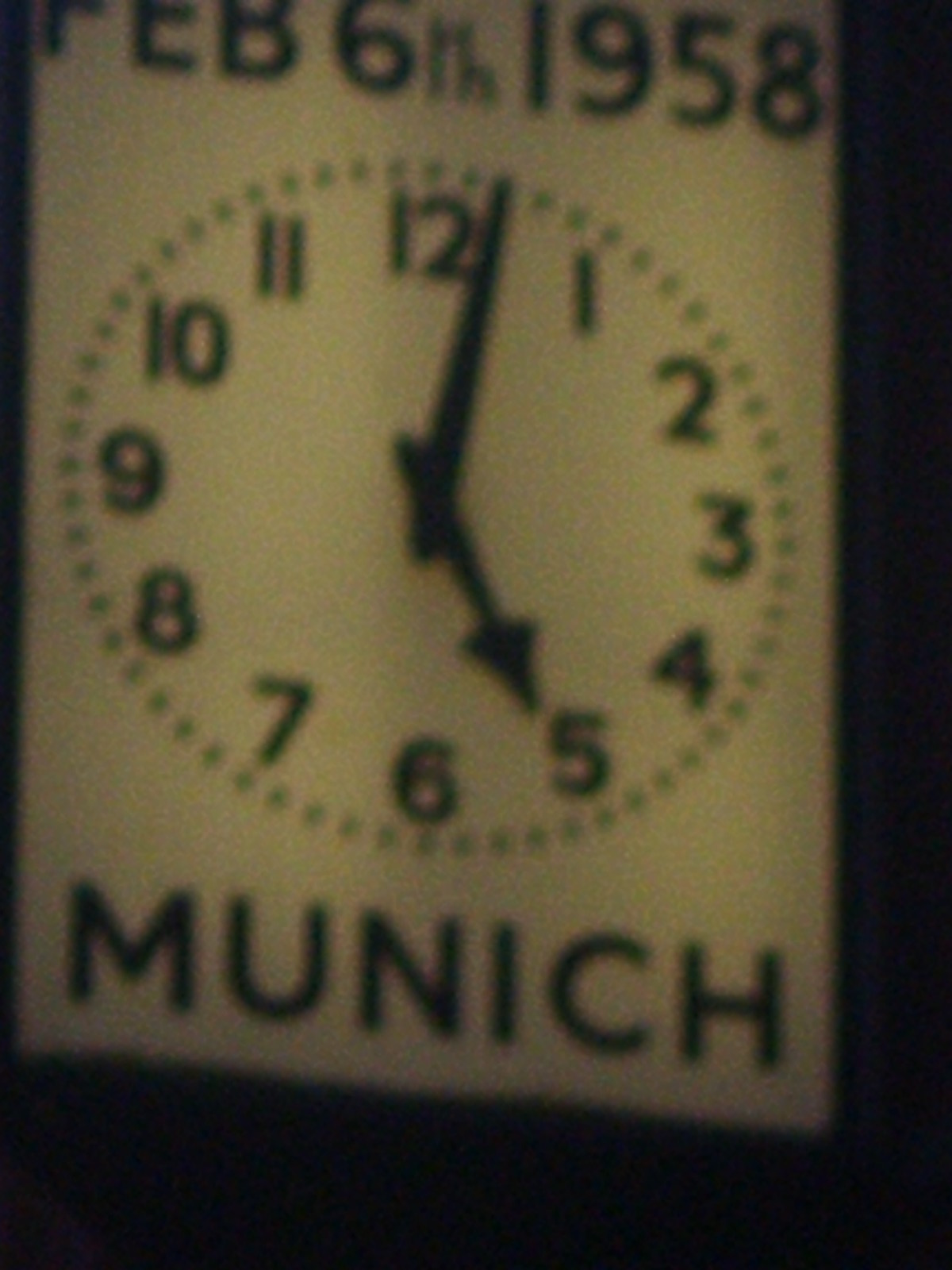This detailed image prominently features a vintage clock situated towards the right-hand side. The clock, framed by a sleek black trim that borders the left and horizontally across the top and bottom by approximately an inch, stands out against the background. The top of the clock face displays the date "February 6, 1958," suggesting either its date of establishment or when the photograph was taken. Below, the label "Munich" is inscribed. The clock itself has a classic design with a pristine white face and bold black hands, showing the time as one minute past five. Encircling the face, black dots form the boundary, adding a distinctive touch. The numerals are also black, ensuring clear legibility and maintaining a consistent monochromatic theme throughout the clock's design.